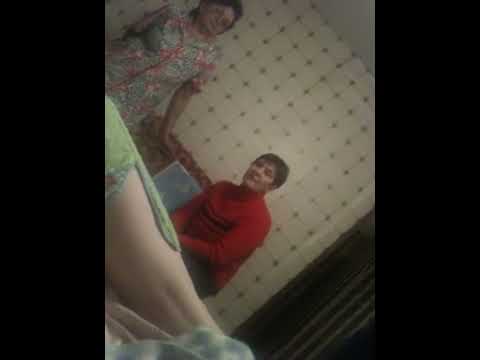This detailed photograph, likely set in a clinical environment such as a doctor’s office or hospital, features two older women against a cream-white tiled wall marked with black dots. The image is framed by vertical black borders on both sides and is slightly tilted to the left. The standing woman, positioned on the left if the image were oriented correctly, wears a green and pink floral dress and glasses, her blackish hair falling to about shoulder-length. To her right, a woman in a red turtleneck sweater and dark pants sits with short, dark brown hair, appearing to be either kneeling or sitting low. Partially visible in the foreground is the pale bare knee of a third person, clad in green pants and lying down with a blanket near their feet, adding to the clinical feel of the scene. The woman in the floral dress steadies herself with her left hand on an unspecified object, while the seated woman gazes towards the person lying down. A dark brown or black door is partly visible on the far right of the image.